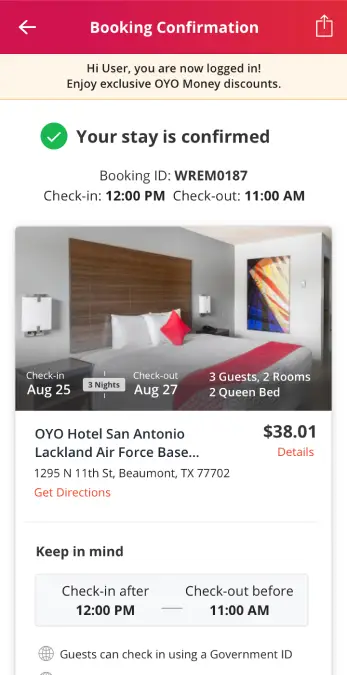This image is a detailed screenshot of a phone screen displaying a booking confirmation for a hotel room. At the top of the screen, set against a red border, there is a small arrow pointing to the left, indicating navigation back. The heading reads "Booking Confirmation," below which a message says, "Hi user, you are now logged in. Enjoy exclusive OYO money discounts."

Beneath this, a green circle with a white checkmark prominently displays the statement, "Your stay is confirmed" in bold text. The booking ID listed is "WREM0187," and key check-in and check-out times are noted as 12 p.m. and 11 a.m., respectively.

Central to the screen's visual content is a photo of a hotel room, focusing on a bed adorned with two white pillows and a smaller red pillow. This bed is flanked by small bedside tables, one of which holds a telephone. A framed photograph hangs on the wall above the bed.

Text above the room photo details essential booking information: "Check-in, August 25, three nights. Check-out, August 27. Three guests, two rooms, two green bed." Below the image, the text specifies the hotel name and location: "OYO Hotel, San Antonio, Lackland Air Force Base" with an address in Beaumont, Texas. The total cost listed is "$38.01," and there is a red "Get Directions" button beneath this.

Finally, at the bottom, a reminder states, "Keep in mind, check-in after 12 p.m. Check-out before 11 a.m. Guests can check in using a government ID," accompanied by a globe icon to the left of the text.